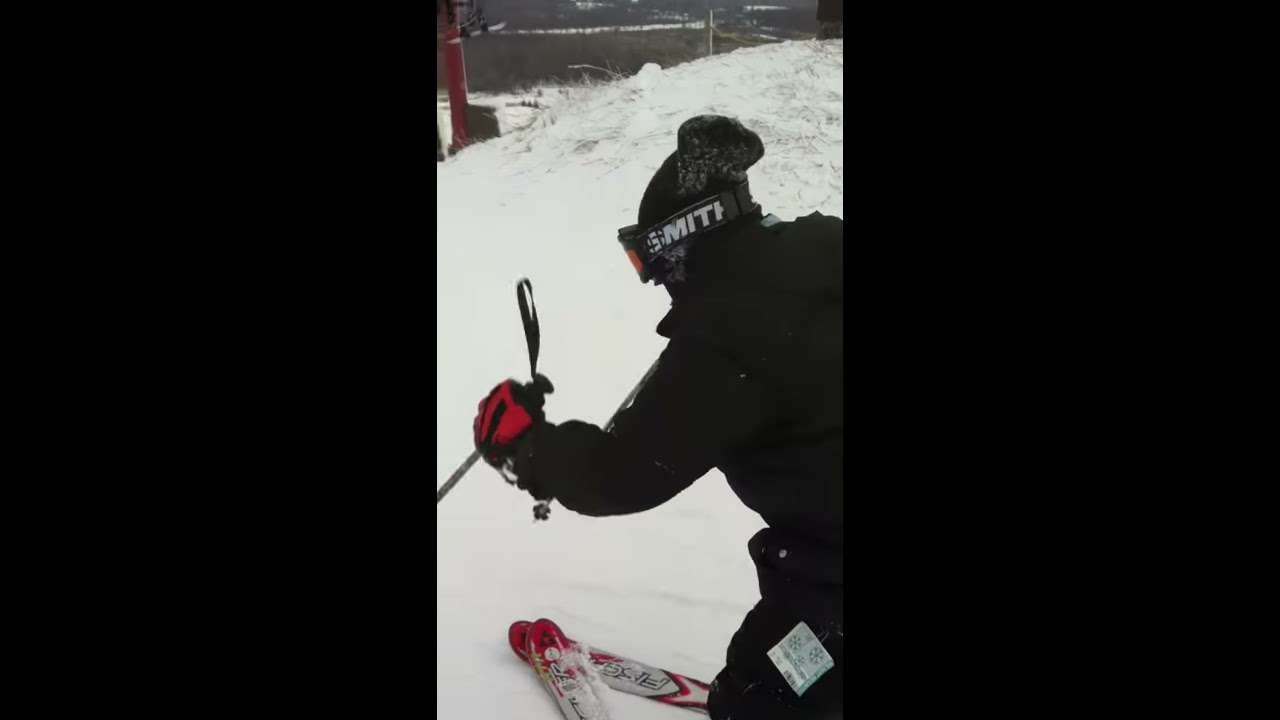In the image, there's a still shot or photograph depicting a skier actively going down a snow-covered ski slope. The central section of the image takes up most of the frame, flanked by two black rectangles that obscure the outer parts of the background. The skier is captured in a vertical highlight within this horizontal rectangular frame, leaning slightly to the left.

This skier, dressed in predominantly black winter attire—including a thick jacket, snow pants, and a beanie—is equipped with red gloves and red skis. The skis are crossed at the front, indicating a slowing motion. They are using black ski poles. The skier also wears black goggles marked with white text spelling "Smith" on the sides.

The background is filled with white, powdered snow enveloping the ski hill, and a wooden fence stretches across the top of the scene. In the upper left corner, a red pole and what seems to be a ski lift are visible, adding context to the outdoor setting during the daytime. The skier’s hat features the letters "M-I-T-I" and a logo, though the finer details of the text on the skis are obscured by snow. The scene illustrates a dynamic moment amid a snowy landscape, emphasizing the skier's movement and the winter environment.